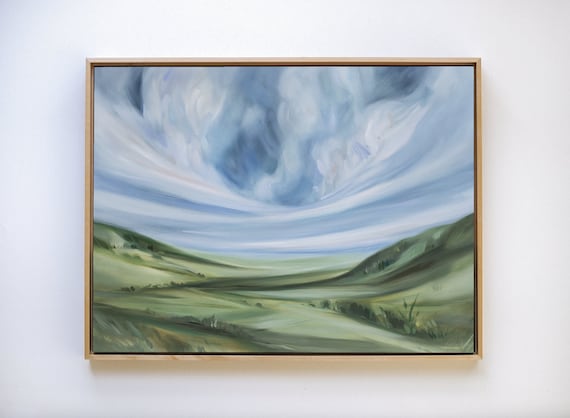This image is a color photograph of a rectangular painting with a landscape orientation, set into a light brown wooden frame featuring a dark brown inner border. Mounted on a plain, smooth white wall under artificial indoor lighting, the painting showcases a surrealistic yet realistic depiction of a sloping green valley that rises to darker green hills on either side. The curved landscape is interspersed with small clumps of vegetation. Above, the sky is filled with thick white clouds that stretch and curl, blending into dark grayish blue tones towards the center, hinting at an impending storm. This detailed artwork combines elements of photographic representationalism with exaggerated curves and surreal sky tones.